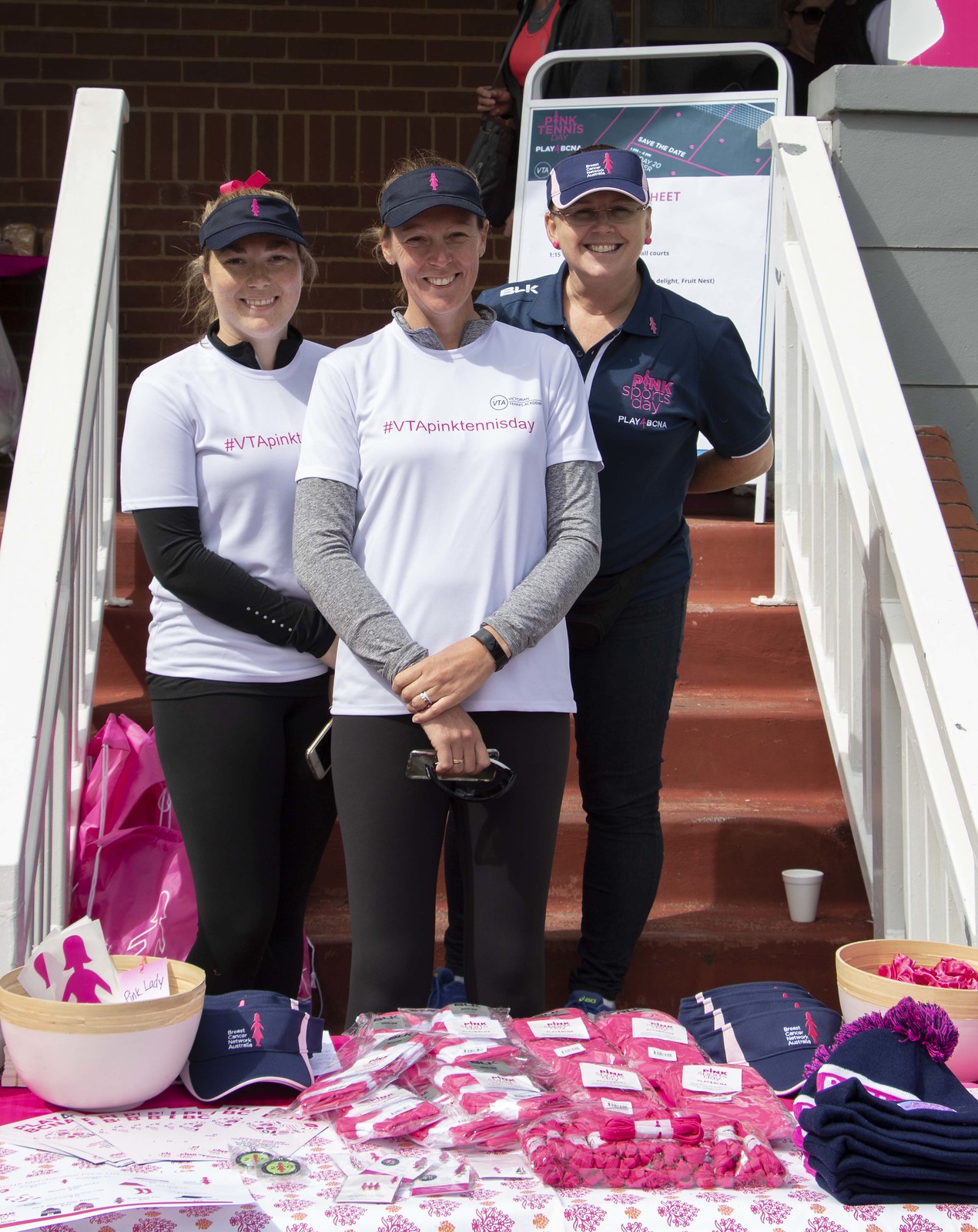The photograph captures three smiling women standing outdoors on reddish-orange steps with white railings. The central figure wears a white T-shirt over a long-sleeved gray shirt and dark pants, along with a navy blue hat featuring red trim. To her left, another woman is dressed similarly, in a white T-shirt over a long-sleeved black shirt and dark pants, also with a matching hat. To her right, slightly behind, stands a third woman in a navy blue polo shirt and dark pants, wearing the same style of hat. Their hair is pulled back, and they all wear expressions of joy. In front of them is a table adorned with various items including blue hats, bowls, and pink items in a baggie. The scene is brightly lit, casting clear shadows across the subjects.